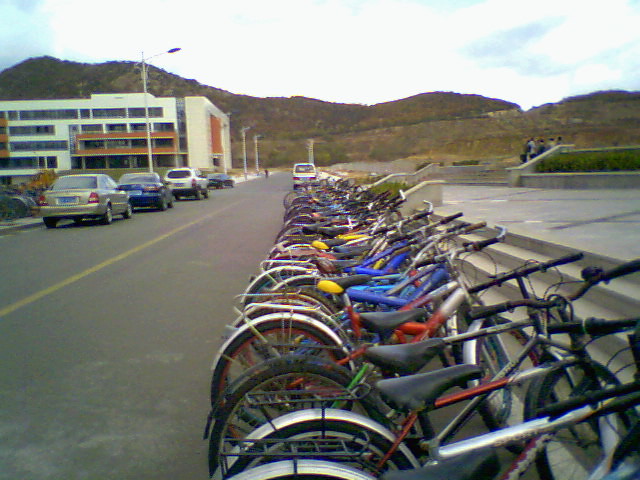The photograph captures an outdoor scene featuring a long and orderly row of parked bicycles, extending from the bottom right to the middle of the image. These bicycles are predominantly uniform in size and style, each equipped with a flat rear rack for carrying items. The bikes, numbering around two to three dozen, come in various colors, including black, red, blue, and yellow.

In the background, a large white and orange five-story building stands to the left, with multiple rows of windows. A clear blue sky with some clouds, along with hills covered in brown and green grass and trees, forms the backdrop. The left side of the image shows several cars parallel parked along the street, while a person can be seen riding a bike on the same street.

On the right side, near the bicycles, there is a large open concrete area with low bushes and planters, along with some concrete steps that lead to another level, where a group of people are gathered, seemingly looking towards the distant hills. The image captures a mixture of urban infrastructure and natural landscape in a setting that seems to be part of a town or city where public bike parking is common. Despite the poor quality and low lighting of the photograph, the detailed elements provide a clear sense of the space and its surroundings.